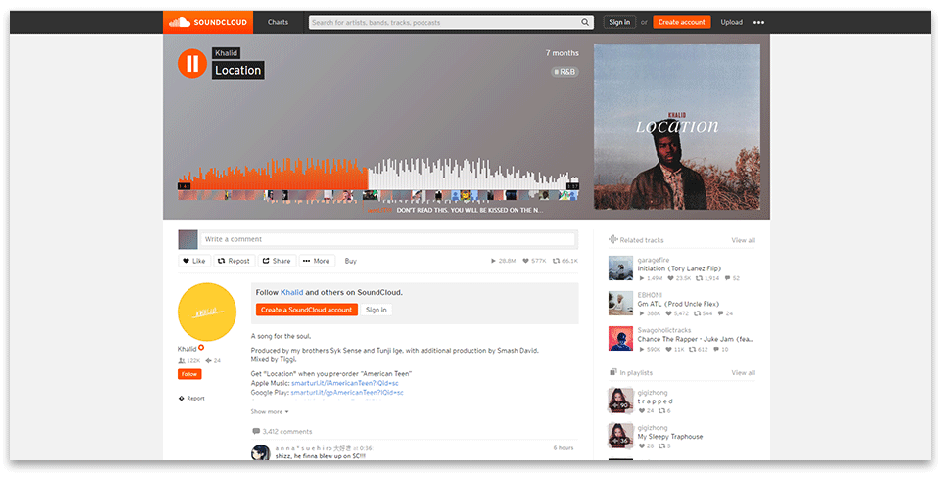The image is a detailed screenshot of the SoundCloud web page, viewed on a laptop or desktop in landscape mode. The top bar on the screen is black, and on the left-hand side is an orange rectangle that features the SoundCloud logo. Next to the logo on the black bar, there is a link labeled "Charts" and a search dialog box with a magnifying glass icon. Towards the right side of the bar, there's a black button that says "Sign In" in white letters and an orange "Create an Account" button with white letters. Further to the right, the text "Upload" is displayed in white on the black bar, followed by a three-dot icon which opens additional options.

Beneath this top bar, on the left side of the screen, there is a pause button depicted within an orange solid circle. To the right of the pause button, it reads "Location," which is the song title, and "Location" is also the artist's name. The text indicates that the song was uploaded seven months ago. Adjacent to this section, there's a small thumbnail of the album cover showing a person standing outdoors against a blue sky backdrop. Below this thumbnail, the text is small and difficult to read but appears to mention something related to the chart position and other details about the song on SoundCloud. Immediately next to this, an orange button invites interaction.

Further to the right of this section, there's a heading that reads "Related Tracks" with a "View All" button nearby. This area displays smaller thumbnail images of album covers from different artists, indicating a selection of related tracks.